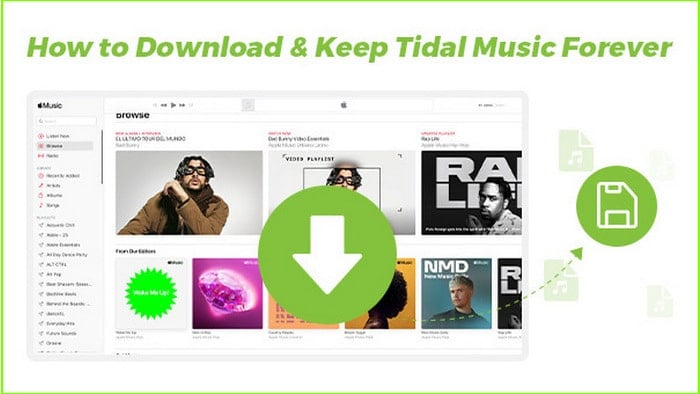A screenshot features Tidal Music, showcasing functionalities similar to Spotify, allowing users to download music. The focal point is the bold, green text that reads, "How to Download and Keep Tidal Music Forever." Overlaying the album artwork in the middle of the image is a white down arrow encased in a green circle, symbolizing the download feature. To the right, a green dotted arrow points towards a disc, suggesting how to save the music. In the backdrop, Apple Music's interface is partially visible, hinting at the possibility of transferring music from Tidal to Apple Music, though no explicit instructions are provided.

In the top-left corner, the Apple Music logo is displayed, with various categories listed beneath it. The currently selected category, though blurry, is situated at the second position. A play button is visible, indicating no active playback. The image showcases two instances of the same individual wearing a brown jacket, glasses, and a brown scarf, indicating a video playlist. Another individual, an African American man, is observed looking at the first figure. 

Below these elements, six album covers are prominently displayed. One album features a green badge, another sports a UFO design, and yet another shows a man with short hair. The background of the image is predominantly white, with special effects including green dotted arrows and a green border that neatly frames the entire scene.